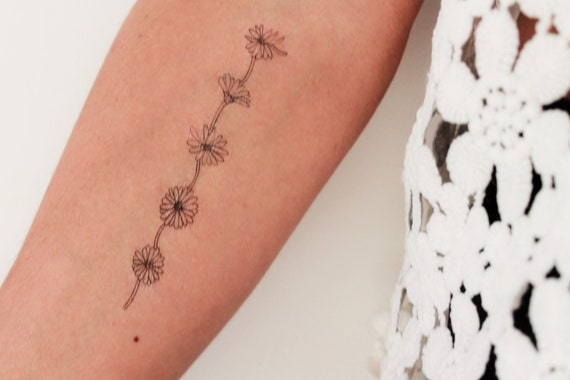The image depicts a close-up view of a Caucasian woman's forearm, showcasing a detailed black ink tattoo. The tattoo features a vertical stalk adorned with five daisy-like flowers, each boasting a multitude of petals and a prominent black center. The flowers mostly face the viewer, except for the second flower from the top, which angles upwards. At the bottom of the arm, there is a noticeable freckle or birthmark. To the right, part of her torso is visible, clothed in a white garment adorned with floral designs and cut-outs, likely a delicate overshirt layered over a darker undershirt. The background of the image is a plain grey wall.